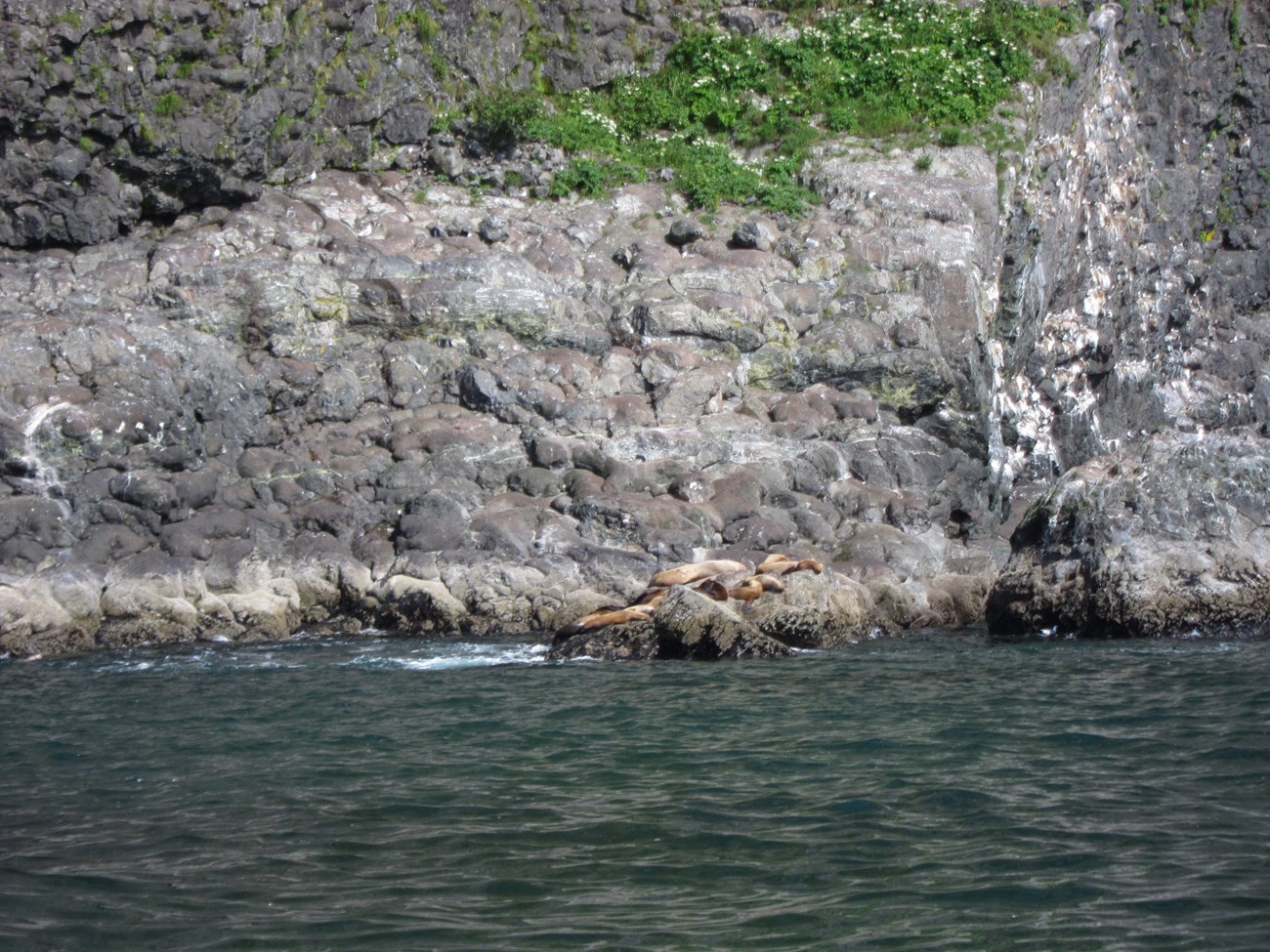The photograph captures a serene outdoor scene featuring a body of water, which could be an ocean, a bay, or a lake, with a slightly wavy, dark greenish-blue hue. In the foreground, several seals, characterized by their light brown, torpedo-shaped bodies, recline on large boulders that jut out from the water, adding a dynamic element to the tranquil setting. The shoreline is met by a sheer rock wall composed of dark gray stones interspersed with white flecks, adding texture and detail to the background. Green plants or vines, adorned with small white flowers, cling to the rock wall, providing a touch of nature’s vibrancy amidst the stony facade. The sunlight reflects subtly off the water’s surface, indicating a sunny day. In the middle ground, white foam forms near the boulders, suggesting the gentle lapping of waves. The image, captured in landscape orientation, embodies a realistic and detailed representation of nature, where the ruggedness of rocks and the peaceful presence of seals coalesce harmoniously.